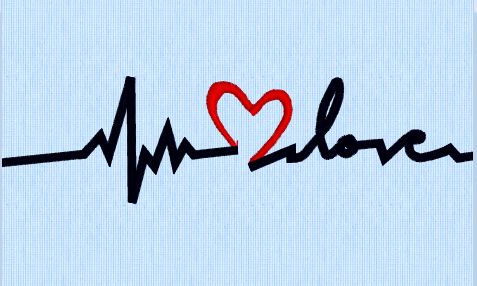The image depicts a detailed, graph-like EKG or heartbeat line that zigzags and fluctuates across the center of a light blue, textured background resembling fine threads or a grid pattern on paper. The line, appearing in very dark blue or black, starts with typical sharp peaks and valleys of a heart monitor. In the middle, it transforms into an open-bottomed, red heart, seamlessly integrating into the heartbeat line. As the pattern continues, the line forms the word "LOVE" in playful, looped and spiked letters, combining elements of the graph. The overall effect is suggestive of an embroidered design, potentially a graphic representation rather than a physical artwork, drawing the eye to its intricate details and balanced use of color and texture.